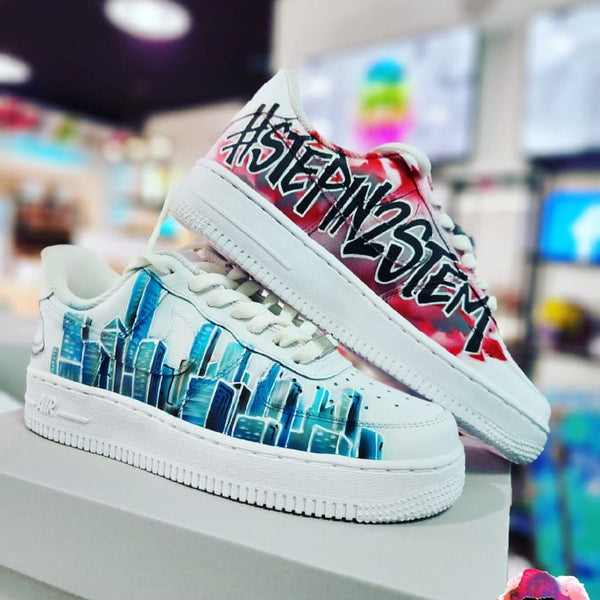The image captures a pair of Nike Air tennis shoes positioned in a retail setting. The sneakers, both with white ribbed soles, are stacked atop a plain white box. The bottom shoe showcases a detailed cityscape design in shades of blue and gray, depicting skyscrapers and various buildings, subtly contrasting against its white background. The top shoe features a striking red, black, and white graffiti-like pattern. Prominently displayed on its side in large black text bordered by white is the phrase "#step into STEM." The photo is taken from the left side, with the background blurred to emphasize the shoes. Blurred elements in the background, such as white walls with various products hanging and black ceilings with white lights, suggest the setting is likely inside a store.